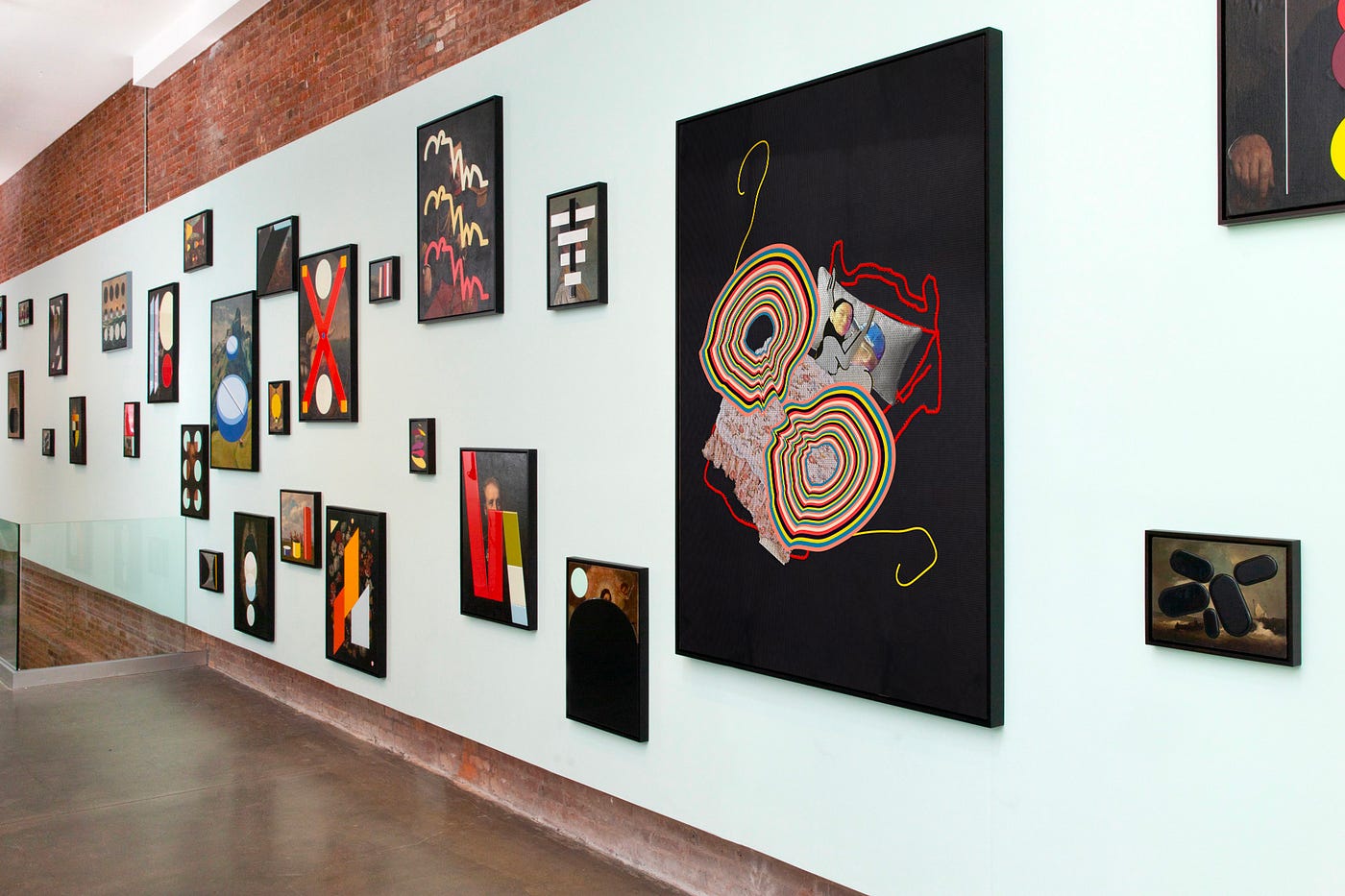The image depicts an art gallery or exhibition space with a prominent brick wall background partially covered by a smooth, white section designed to display numerous artworks. The floor is hardwood with brown trim, adding a classic touch to the modern setting. At the far left, there's a glass partition suggesting a downstairs area. The wall showcases around 20 to 30 pieces of art, ranging from small to large, positioned in a seemingly random yet captivating arrangement.

The most noticeable piece on the right features a large black canvas with a red outlined bed occupied by two stylized figures, likely a couple, adorned with vividly colored circular shapes resembling yarn. Above this piece, whimsical multi-colored patterns suggest a burst of creativity. 

Overall, the displayed artworks lean towards abstract expressionism with a variety of vibrant shapes and lines, conveying different moods and themes. The ceiling overhead is white, contributing to the bright and inviting atmosphere, while the perspective of the image captures the depth and dimension of the gallery space, guiding the viewer's eye from the closest artworks on the right to those disappearing into the distance on the left. The overall ambiance is one of artistic exploration and contemporary aesthetics.